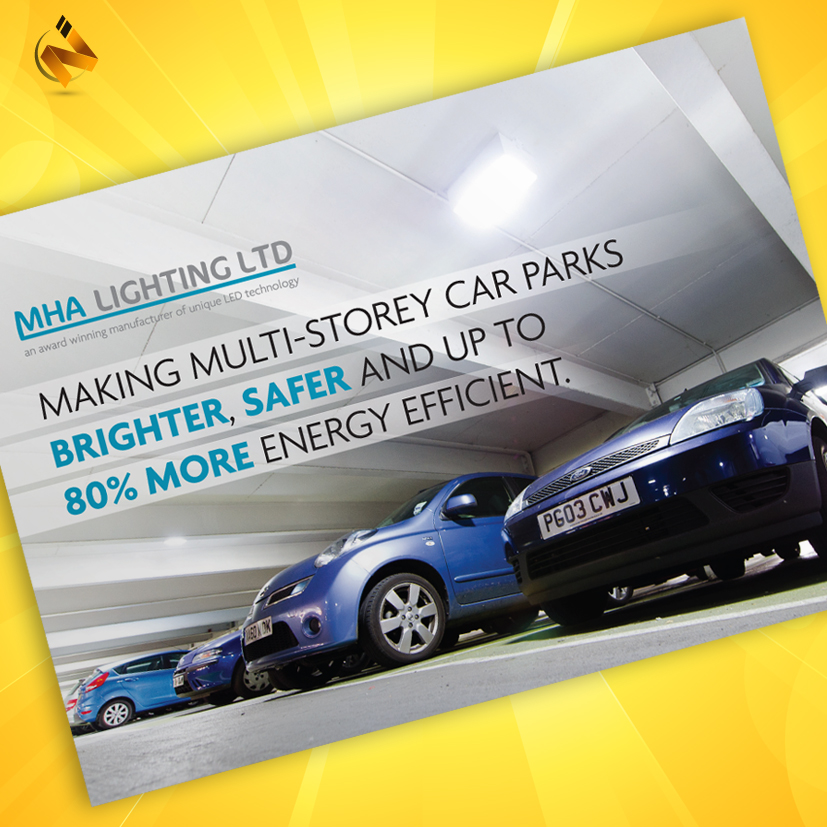In the image, a yellow rectangle prominently displays the text "MHA Lighting LTD" underlined, with the tagline "Making multi-story car parks brighter, safer, and up to 80% more energy efficient." The words "brighter," "safer," "80% more," and "MHA" are highlighted in blue. Below this, several cars are parked in a lot, featuring predominantly blue vehicles. Some cars are parked head-in while others are backed in. Notably, the license plate on the last car reads "PGO 3CWJ."